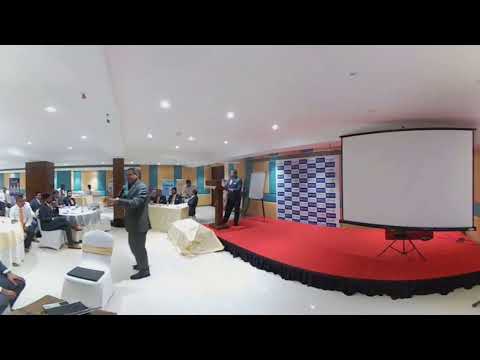The image depicts a large, open conference room with white tile flooring and white ceilings featuring several circular spotlights. The room is dominated by a red stage positioned on the right side, adorned with black curtains and a large white screen, currently unlit. Behind the stage podium, a wall displays a blue and white checkered pattern. A dark-skinned man in a blue shirt and black pants stands behind the podium, while to his left, a long table with a white tablecloth holds several men in suits.

In the center of the room, a dark-skinned man with gray hair, dressed in a gray business suit and black shoes, holds a microphone as he addresses the seated audience. The attendees, predominantly men in business suits, are seated at round tables draped with white tablecloths. Scattered drinks are visible on the tables. The walls behind the audience feature alternating yellow and green stripes, adding a splash of color to the otherwise professional setting. The detailed and organized room setup, along with the business attire of the individuals, suggests that a formal conference or meeting is taking place.